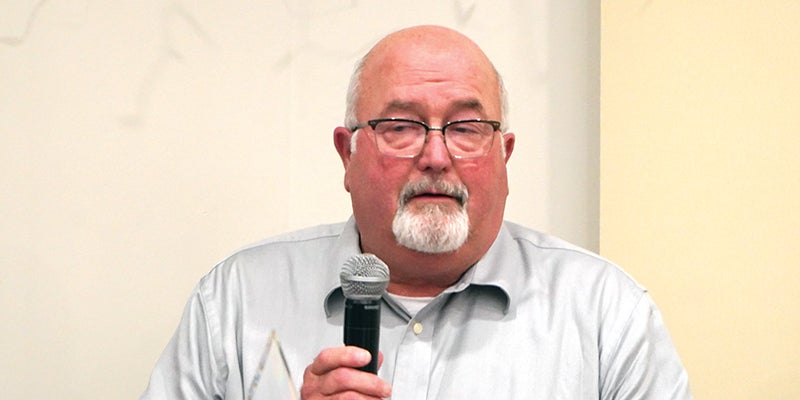In this detailed photograph, a middle-aged, slightly heavyset man is prominently centered and shown from the chest up, with his lower body cut off at the bottom of the image. He has a large, round face with a bald top and a fringe of white hair on the sides. His facial hair consists of a mostly white, slightly gray goatee and mustache. The man wears black-framed eyeglasses and is dressed in a light-colored button-up shirt—either light blue or gray—with the top button undone, revealing a white T-shirt underneath.

His right hand is raised in front of his chest, holding a black-handled microphone with a silver end, with his forefinger and middle finger visible over the front of the microphone. The background features a light pink wall with a vertical gray stripe visible over his left shoulder, creating a contrast with the slightly darker pink wall to the right of the stripe. The man's gaze is slightly to the left, suggesting he might be addressing an audience or speaking at an event.